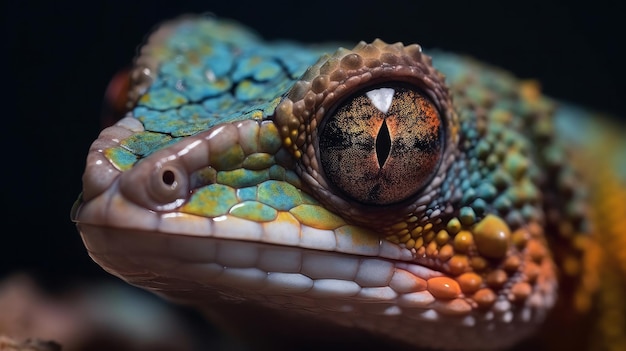The image is a close-up photograph of a colorful gecko's head, sharply detailed against a black background. The gecko's eyes are particularly striking, featuring a black, seed-shaped slit at the center, surrounded by radiant hues of brown and orange. The scales on its head exhibit a vibrant array of colors: shades of blue and orange predominate, with white scales under its mouth and along the chin and nostrils. The nostril on the left side of the gecko's head is clearly visible, punctuated by smooth, white scales. The side of its head also showcases a prominent yellow protrusion and some orange scales. The area around the eyes is adorned with spiky scales, leading from the bulging eyes down to where the cheek meets the eye. The smooth, white coloring of the gecko’s nose contrasts with its richly patterned and textured head, creating a captivating mosaic of colors and textures.